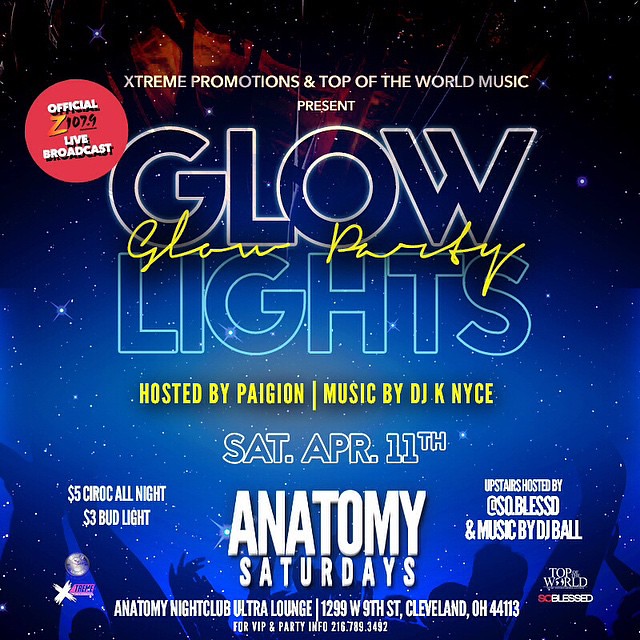The promotional poster for the music event, "Glow Lights Glam Party," features a striking design of a night sky, transitioning from black to lighter blue, adorned with stars. Organized by Extreme Promotions and Top of the World Music, and hosted by Pagon, the event boasts music by DJ K Nice. The central text, outlined in white, prominently lists "Glow" and "Lights," with "Glow Party" elegantly scripted in yellow between them. An additional highlight is an Official 107.9 Live Broadcast, marked by a red circle with white lettering. Scheduled for Saturday, April 11th, the party at Anatomy Nightclub Ultra Lounge (1299 W 9th St, Cleveland, OH 44113) promises $5 Ciroc all night and $3 Bud Light. Upstairs, At So Blessed with DJ Ball hosts another segment. VIP and party details can be accessed via 216-789-3492. The bottom of the poster features silhouettes of a crowd with their hands raised, evoking a concert atmosphere.